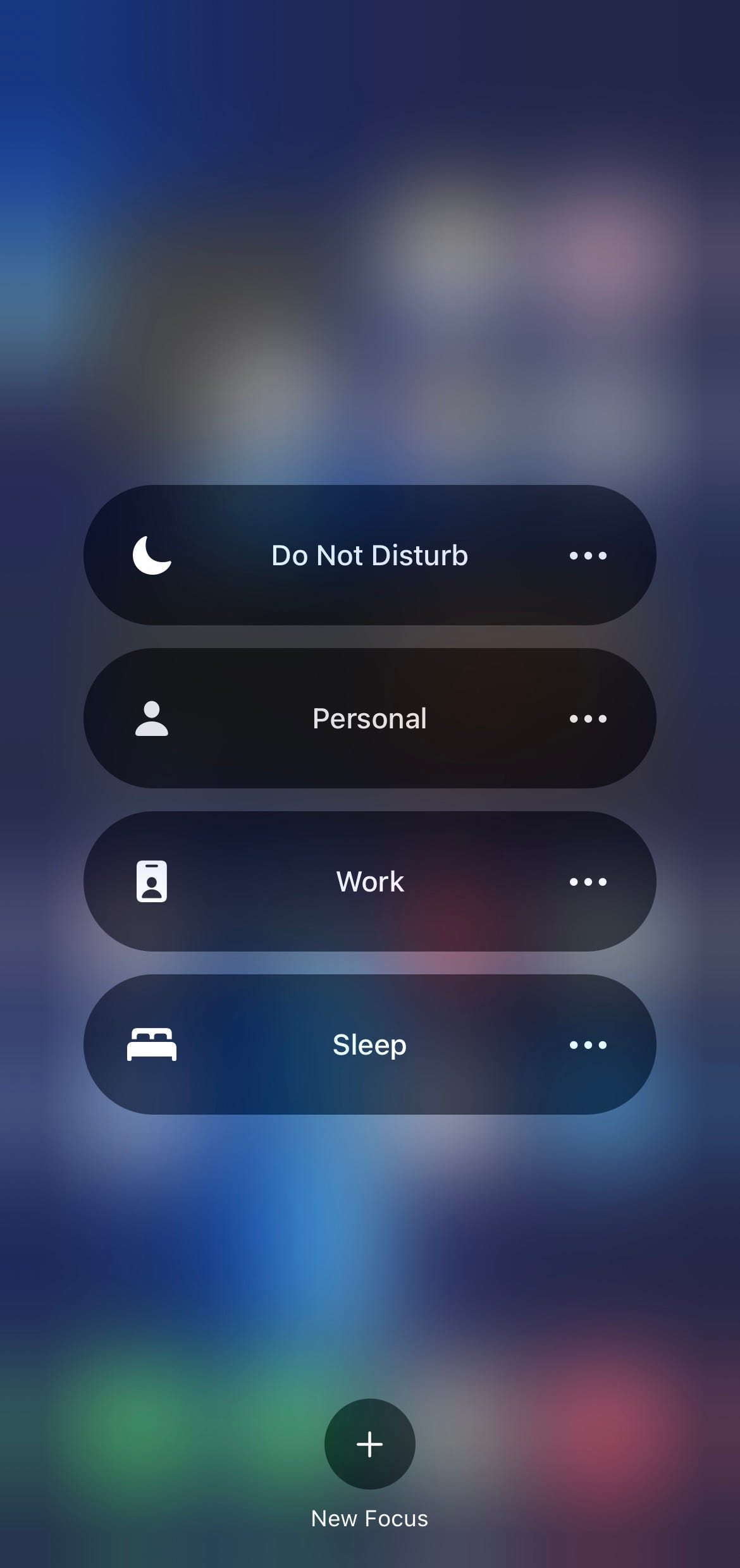The image depicts an iPhone screen with the Control Center interface visible after swiping down. At the top, there is a "Do Not Disturb" option accompanied by a crescent moon icon. Below are categorized sections labeled as "Personal," "Work," and "Sleep," each marked with a specific icon: a person, briefcase, and bed respectively. Each category has a menu button represented by three vertical dots, allowing for additional options.

The text for all these categories is displayed in white against an overlay of dark, semi-transparent black shapes. Behind this overlay, the blurred background reveals the user's home screen, with app icons faintly visible. At the screen's bottom, prominent icons suggest the phone and message apps, shown in green and white respectively, typical of the iPhone's dock apps layout. Additionally, a plus button labeled "New Focus" is present at the bottom, inviting the user to create a new focus mode. Among the blurred icons, the Notes app is distinguishable by its yellow and white color scheme.